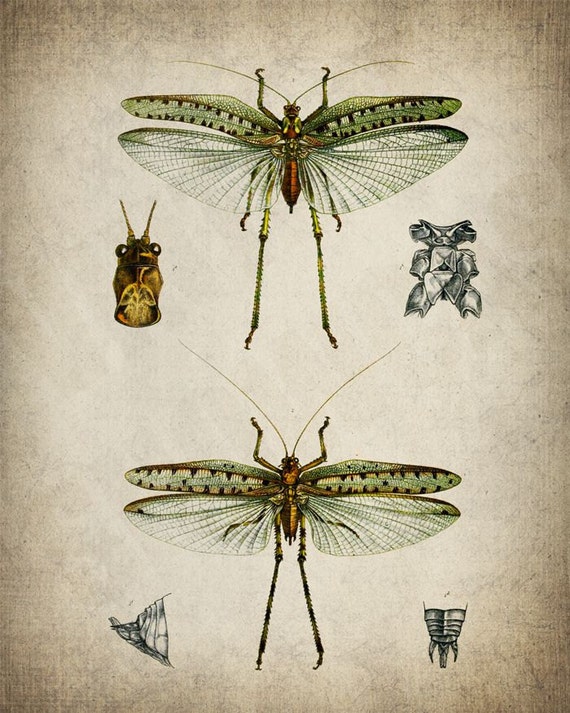The image composition showcases an insect against a light tan background. At the top of the frame, there is a vivid green grasshopper, characterized by its long, slender legs and extended wings. This grasshopper also features an exceptionally long antenna. Toward the bottom of the image, another view of the grasshopper reveals slight brown colorations on its upper body, maintaining the same long antenna, legs, and wings. Positioned centrally, a close-up captures intricate details of the grasshopper's body parts, including its head, tail, and back, providing a comprehensive perspective of its physical attributes.